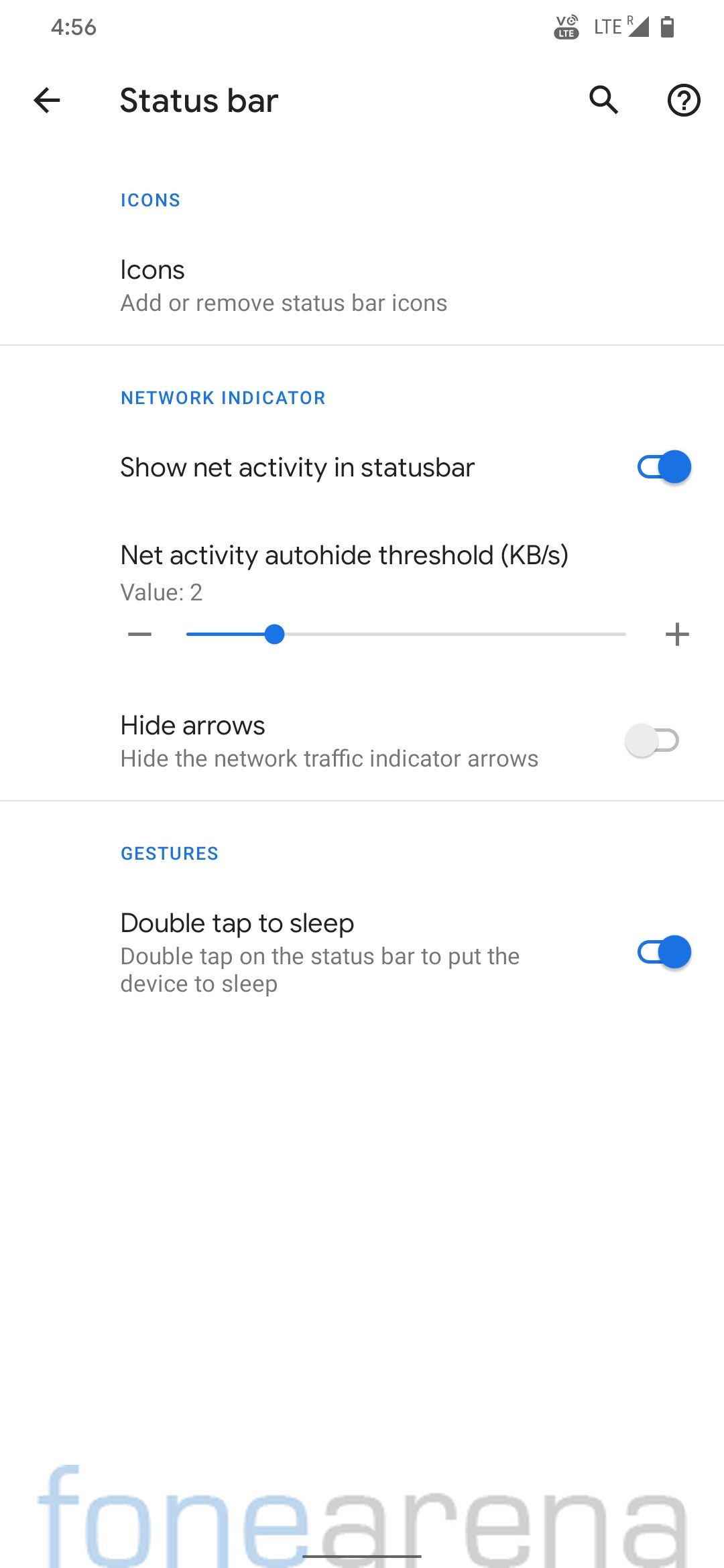The screenshot appears to be from a smartphone's settings menu. The time displayed is 4:56, and the status bar shows an LTE connection and a battery level at approximately 75%. The image highlights the "Status Bar" settings, specifically focusing on the icons and network activity indicators.

The first section is titled "Icons" and provides options to add or remove icons from the status bar. The "Network Indicator" is enabled, displaying network activity in the status bar. The "Net Activity Auto-Hide Threshold" is set to 2 kilobytes, and the option to "Hide Arrows", which would conceal network traffic indicator arrows, is turned off.

In the "Gestures" section, the "Double Tap to Sleep" feature is enabled, allowing users to put the device to sleep with a double tap gesture.

The bottom of the screenshot includes a watermark reading "PhoneArena," stylized as "FoneArena".